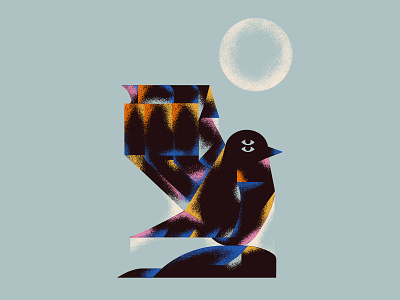In this abstract artwork, set against a teal-gray background, a black bird assembled from geometric shapes including squares, rectangles, and triangles takes center stage. The bird is accented with vibrant splashes of orange, pink, yellow, and blue at the corners and edges of these shapes. Uniquely, it features two eyes positioned one above the other on the side of its head, enhancing the abstract feel. Above the bird, a large white moon fades to gray at its center, casting a calming glow. Behind the bird, an angled rectangular structure with similar colorful accents extends from its body, resembling a tilted milk carton, which adds an additional peculiar, yet harmonious, bird-colored shape to the scene.